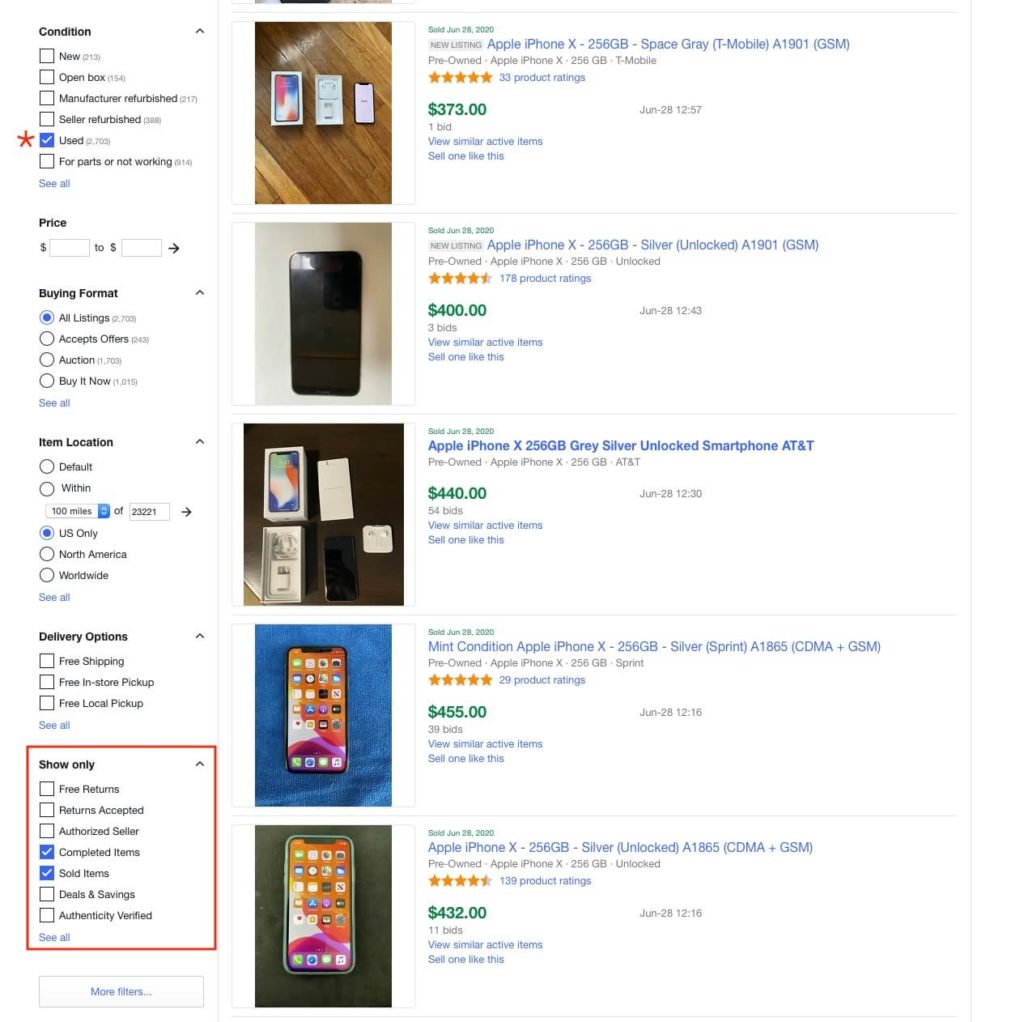This image captures a webpage from a shopping website displaying a list of used Apple iPhones available for purchase. The left-hand column of the webpage contains various filter options, including "Condition," "Buying Format," "Item Location," "Delivery Options," and "Show Only." The "Show Only" section, located at the bottom left-hand corner, is prominently highlighted with a red-outlined box.

The main section of the webpage showcases five separate listings for Apple iPhone X models, each accompanied by a photograph of the item situated to its left. The listings are as follows:
1. Apple iPhone X 256GB Space Gray (T-Mobile)
2. Apple iPhone X 256GB Silver (Unlocked)
3. Apple iPhone X 256GB Gray/Silver (Unlocked Smartphone, AT&T)
4. Mint Condition Apple iPhone X 256GB Silver (Sprint)
5. Apple iPhone X 256GB Silver

Each iPhone listing is enclosed within a thin gray box and highlights key details in green, specifically the price each item has sold for, emphasizing the "Completed and Sold Items" filter. Notably, the "Condition" filter has the "Used" checkbox selected, and the "Buying Format" filter is set to display "All Listings." Additionally, the item location filter is set to "US Only," ensuring that all displayed items are from sellers within the United States.